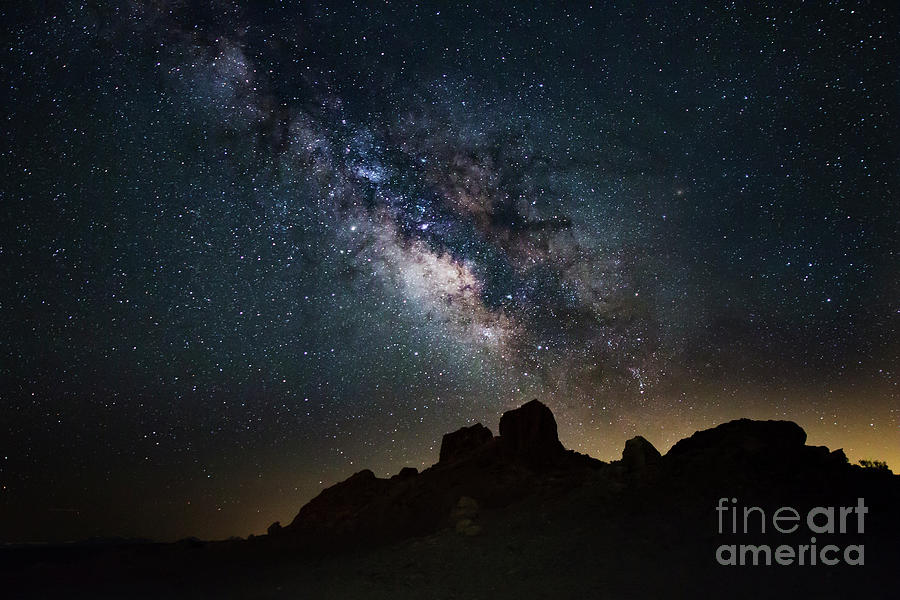This photograph, credited to Fine Art America with their logo faintly inscribed in light gray at the bottom right corner, captures a mesmerizing night sky. Dominating the scene is a rich tapestry of thousands of stars scattered across a dark blue expanse. The center of the image is particularly striking, showcasing what appears to be the Milky Way or another galaxy, characterized by a swirling, rippled appearance with dark interstellar dust contrasted by lighter, white and gray, cloud-like formations. Below this stellar display, the bottom right features a silhouetted rocky formation or mountain peak, partially illuminated by a subtle aura of orange-yellow light. The overall image beautifully balances the serene, star-speckled sky with the rugged, dark silhouette of the earth, creating a captivating visual of celestial wonder and terrestrial mystery.